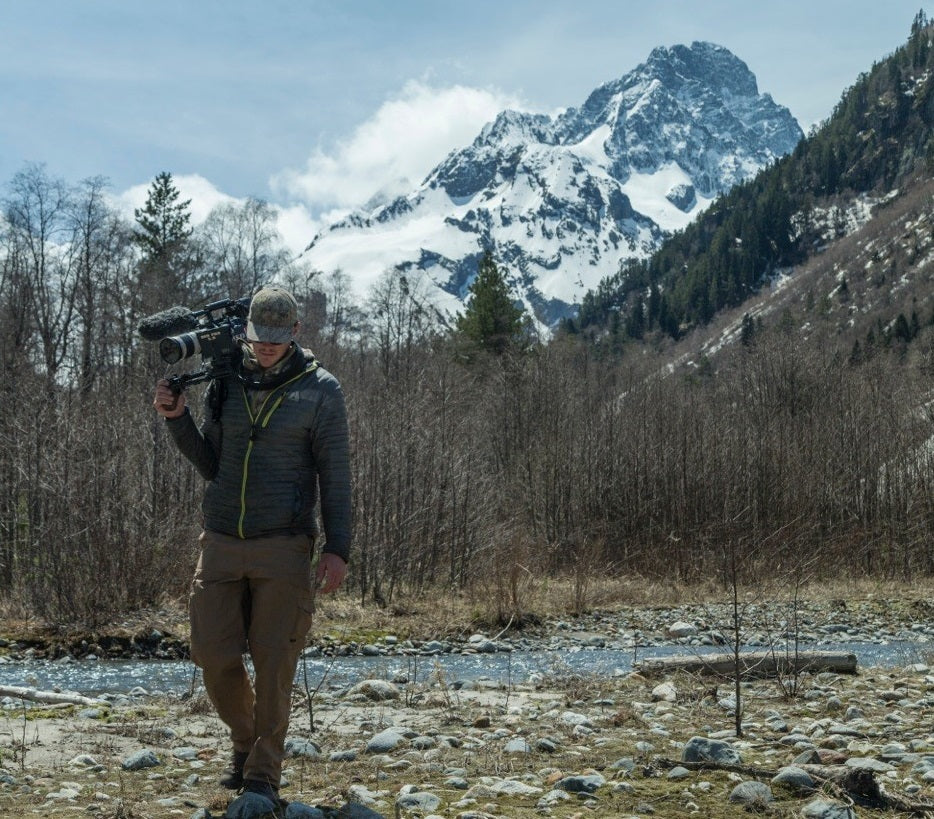The photograph captures an expansive winter landscape featuring grayish-blue, snow-capped mountain ranges under a mostly blue sky adorned with a few white clouds. The foreground is dominated by a small body of water, likely a lake or pond, surrounded by light green grass and scattered rocks. The terrain extends into spindly, light brown trees, some bare and others thinly cloaked in greenery, leading up to the snowy mountains. In the midground, you can discern patches of evergreens ascending the mountain's right slope. To the left of the frame, a man stands on rocky ground near the water, wearing a gray jacket with a yellow stripe, a gray cap, and dark brown cargo pants. He appears to be a photographer, holding a video camera over his right shoulder. Nearby, a log rests among the gray rocks, adding to the rugged natural setting.